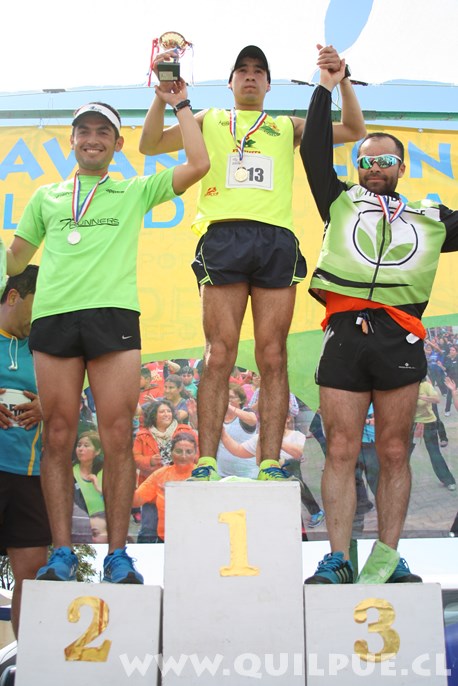This color photograph captures the first, second, and third place winners of an unknown competition, all adult males, standing on podium blocks. The blocks, which are light gray with gold numbers (1, 2, and 3), have the number one block taller and center stage. 

In the middle, on the tallest podium marked number 1, stands the first-place winner wearing a yellow sleeveless shirt, blue shorts with yellow trim, and light green shoes with blue shoelaces. He has a red, white, and blue lanyard around his neck with a gold medal at the end and both arms raised in celebration.

To his left is the second-place winner, on the podium marked number 2, dressed in a lime green short-sleeve shirt, black Nike shorts, and blue shoes. He has a similar gold medal lanyard and is wearing a white visor. He is smiling and holding up his right hand.

On the right, on the third-place podium marked number 3, stands the third-place winner in an orange shirt with a blue or green vest, black shorts, and blue shoes. He is wearing mirrored sunglasses that reflect blue light and has a gold medal lanyard around his neck. He holds his left hand up.

Behind the winners is a backdrop depicting a large crowd, although it appears to be an image rather than an authentic crowd. A giant scroll hangs above them in the backdrop, and a web address, www.quilpue.cl, is visible at the bottom of the image. All three winners are facing forward with arms raised, exuding a sense of achievement and celebration.